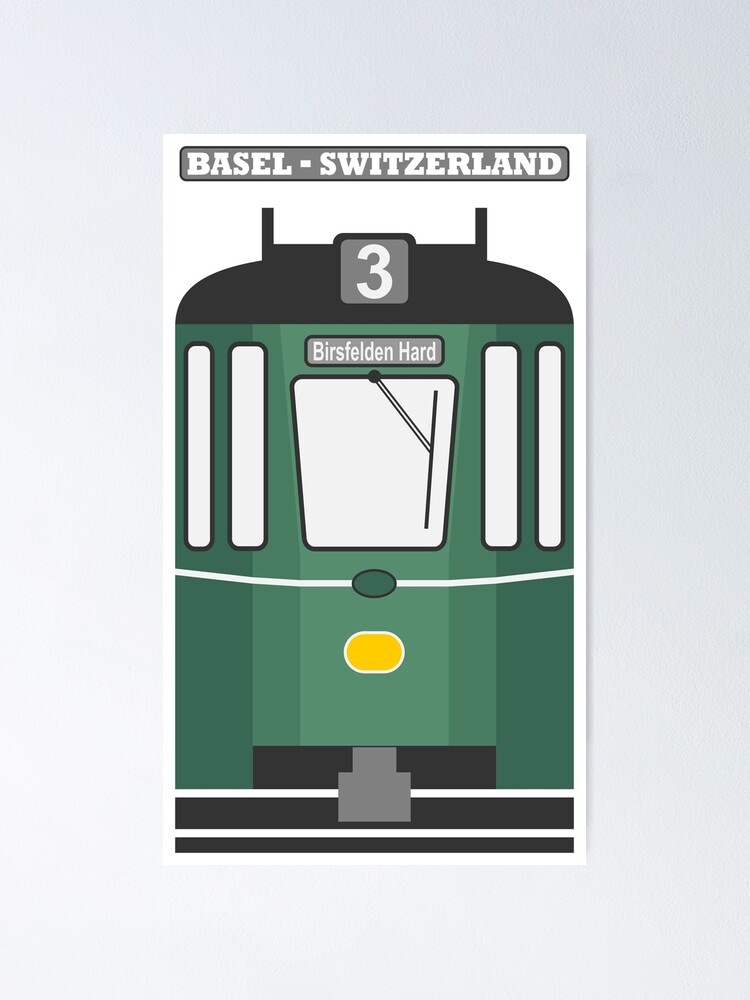The photograph is a product image intended for online commercial listings, featuring a rectangular poster with a light gray background, evocative of a wall. The poster itself is white and rectangular, with its height twice the width. At the top, there is a gray rectangular banner with white text reading "Basel-Switzerland." Below this, the poster showcases a cartoon-style drawing of a green tram or trolley facing forward. The tram has five windows on the front, with the center window featuring a drawn windshield wiper. The tram's roof is black, and it bears the number "3" in white font on a gray background. Above the driver's window, there is a street name, "Versfeldenhard." The front of the tram also includes a yellow oval, likely depicting the headlight, and a green circle beneath it. Additionally, two black bars protrude from the roof, presumably representing the connectors to overhead power lines. The overall design suggests a vintage-inspired advertisement or signage for the tram system in Basel, Switzerland.